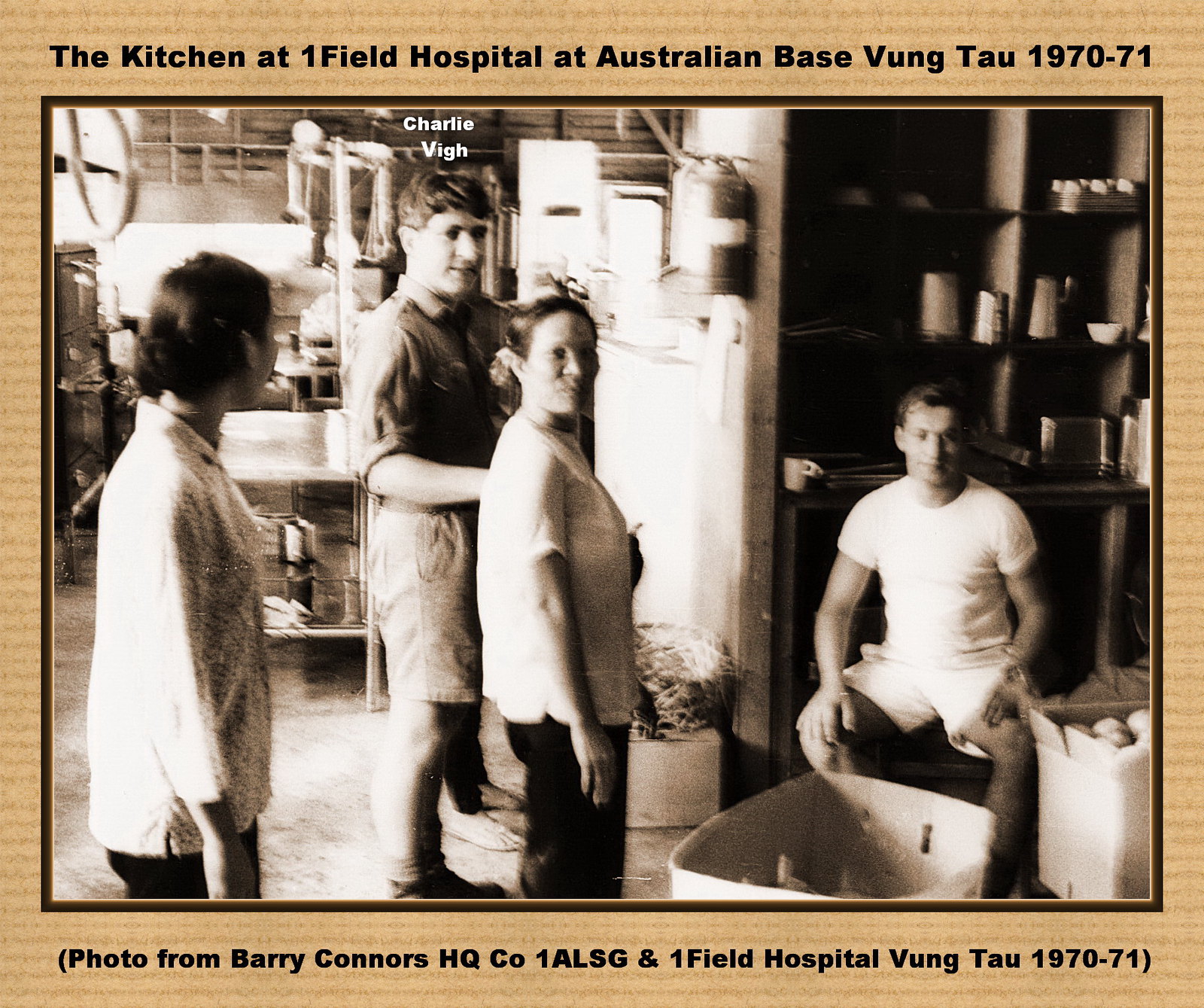The black and white historical photo, captioned at the top as "The Kitchen at Onefield Hospital at Australian Base, Vung Tau, 1970-1971," captures a moment from a military kitchen setting. Below the image, it notes, "Photo from Barry Connors, HQ Co., One ALSG and Onefield Hospital, Vung Tau, 1970-71." In the photo, there are four individuals: two women and two men. Positioned in the center, a middle-aged woman gazes directly at the camera, while an Asian woman to her left looks away towards the two central figures. Standing behind the middle-aged woman is a Caucasian man, presumably with brown hair, identified as Charlie Bigh. To the far right, another Caucasian man sits in a chair with a laundry basket—possibly containing onions or potatoes—in front of him. The backdrop of the photo reveals kitchen paraphernalia, including shelves, pans, muffin trays, and large circular tins, providing a glimpse into the kitchen operations during the early 1970s at this military base.